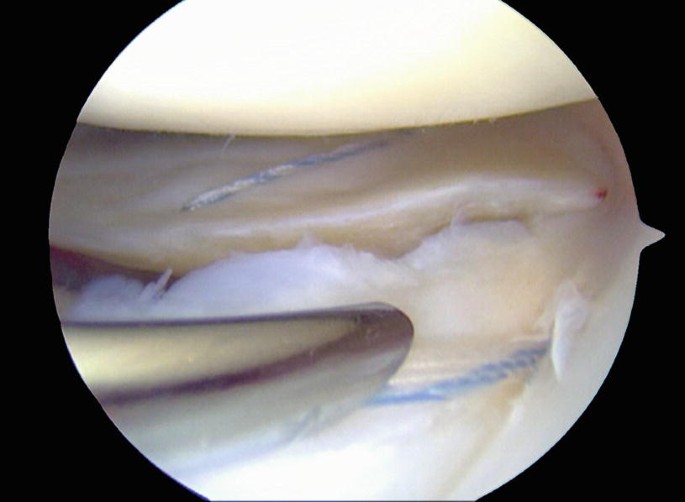This image showcases a circular, microscope view of a distinct, swirling, and layered texture that strongly resembles bone or teeth. The dominant colors are dark grayish-brown with white interspersed throughout, creating a striking contrast. On the top and bottom edges of the circular frame, the image is predominantly white, emphasizing the central bone-like structure. The background beyond the circled view is pitch black, further focusing attention on the intricate details within the circle. A subtle metal instrument, slightly curved, protrudes from the lower left side, curving downward onto the white structure. Additionally, thin white and blue twisted elements, resembling wiring, are noticeable against the white background, adding to the image's complexity. The overall presentation evokes the appearance of a planet floating in space, with its intricate textures and layers, creating a visual intersection of art and science.